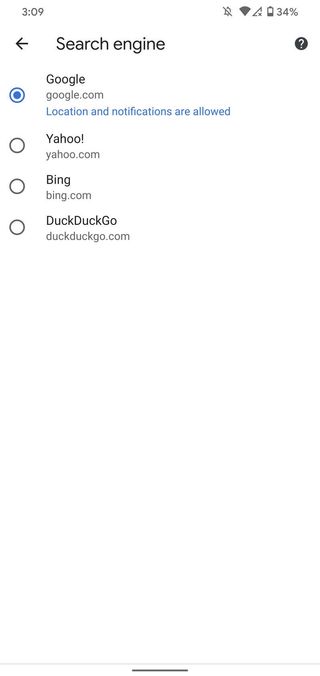A detailed screenshot of a smartphone setup page showcases the user configuring their search engine preferences. The top portion of the screen displays essential phone status icons: the time on the left, a silenced notification bell icon, a strong Wi-Fi signal, disabled mobile data indicated by an "X," and a battery level sitting at 34%. An arrow pointing left precedes the bold, black text "Search Engine," which is highlighted prominently. Adjacent to this is a black circle containing a white question mark, presumably for help or additional information.

Below the header, four circle options are listed for selecting a preferred search engine. The first circle, highlighted in blue, indicates the current selection, labeled "Google, google.com," with permissions for location and notifications enabled. The other three options are "Yahoo, yahoo.com," "Bing, bing.com," and "DuckDuckGo, duckduckgo.com," each with their respective URLs, but none currently selected.